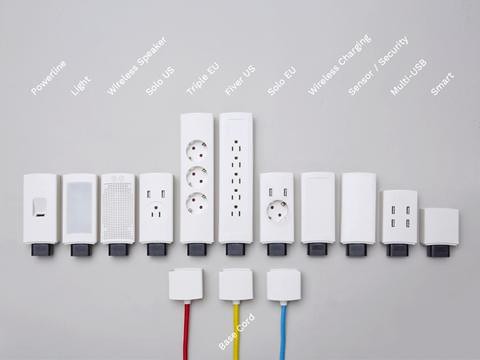This detailed image, likely a digital illustration or advertisement, features a light gray background and displays a variety of power strips and wall sockets labeled in white text. The power strips are aligned across the center of the image in an organized manner, with their sizes varying from small to large. The middle section holds the tallest strips, one featuring three outlets, another with four, and a smaller one with two outlets. Each power strip is white with a black base, showcasing different plug types from around the world.

The labels floating above each power strip indicate their usage, including terms like "power," "light," "wireless speaker," "USB," "wireless charging," "sensor," and more. At the bottom of the image, three small white square blocks, each with a colored cord extending downward, are prominently displayed. The cords are red, yellow, and blue, with the label "bass cord" positioned above them. These elements together convey a detailed visualization of a range of international power solutions and their respective connections.